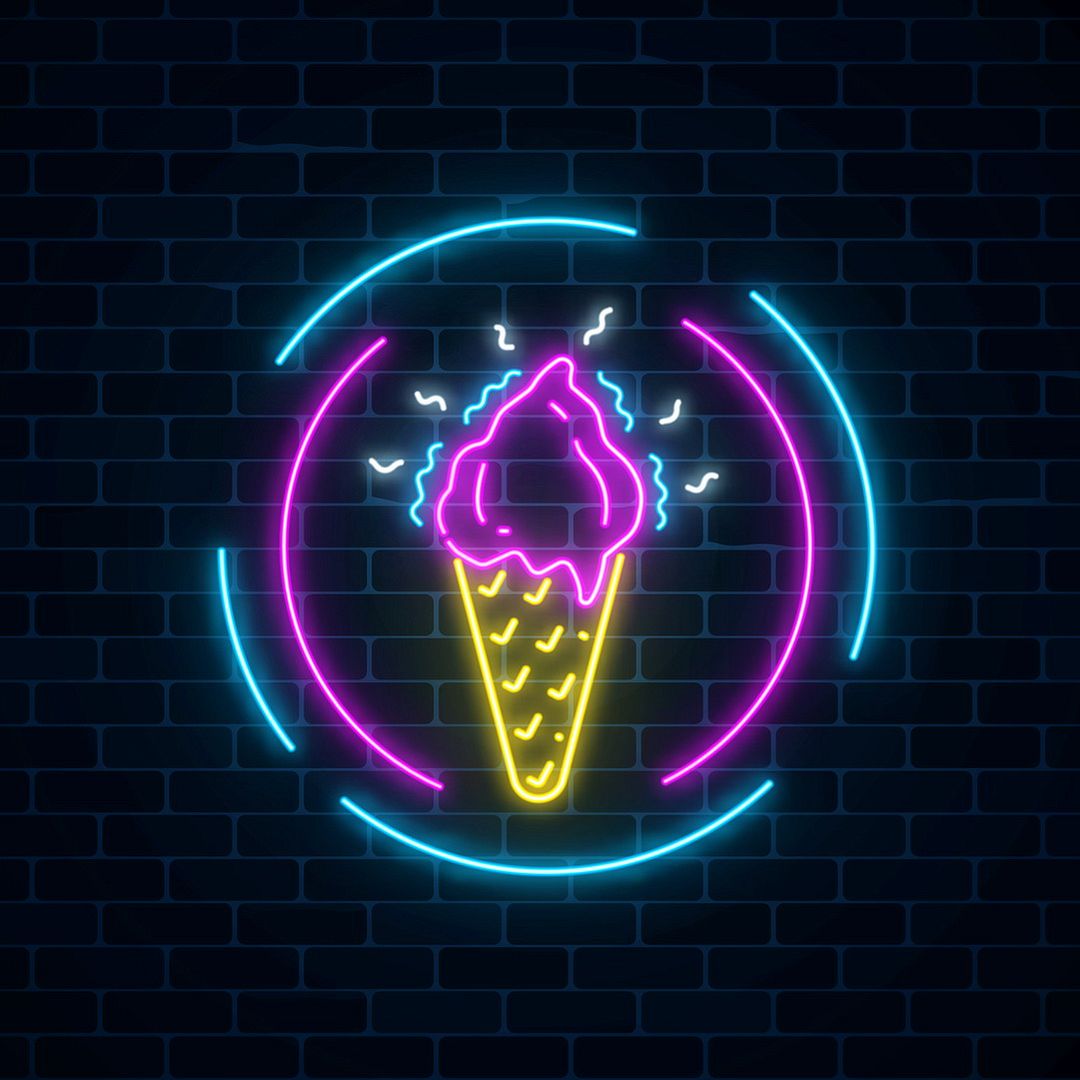The image depicts a neon sign of an ice cream cone mounted on a black brick wall, with blue grout lines in between the bricks. The cone is outlined in yellow neon and has a rounded bottom, visually similar to a sugar cone texture. Atop the cone, there's a hot pink scoop of ice cream, with blue sprinkles adorning its surface, and radiating white sprinkles that suggest coldness. Surrounding the ice cream are two pink neon arcs on the left and right, further encircled by four blue arcs that almost form a complete circle, with the lower-left segment being noticeably smaller. This intricate neon artwork captures the essence of a delightful ice cream treat, with its vibrant colors and dynamic, radiant design.